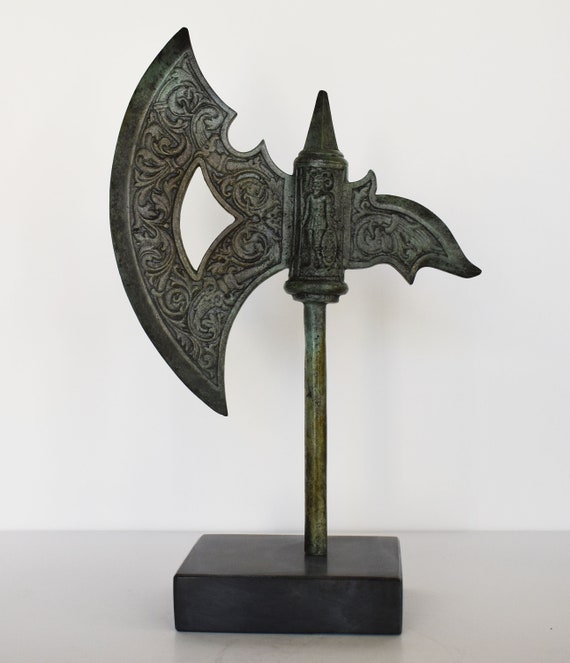This image showcases an ancient artifact weapon, prominently displayed against a white background. The weapon features a detailed, sharp axe head attached to a green and brown metallic rod. The axe head, likely historical and possibly used in battle, has intricate engravings along its surface, including patterns of swirls, curves, and a depiction of a human-like figure near the top of the handle. The blade curves into a half-circle with a distinct triangular opening in the center. This artifact is secured on a flat, square black base, which might be wooden or plastic, allowing it to stand upright and be fully visible.